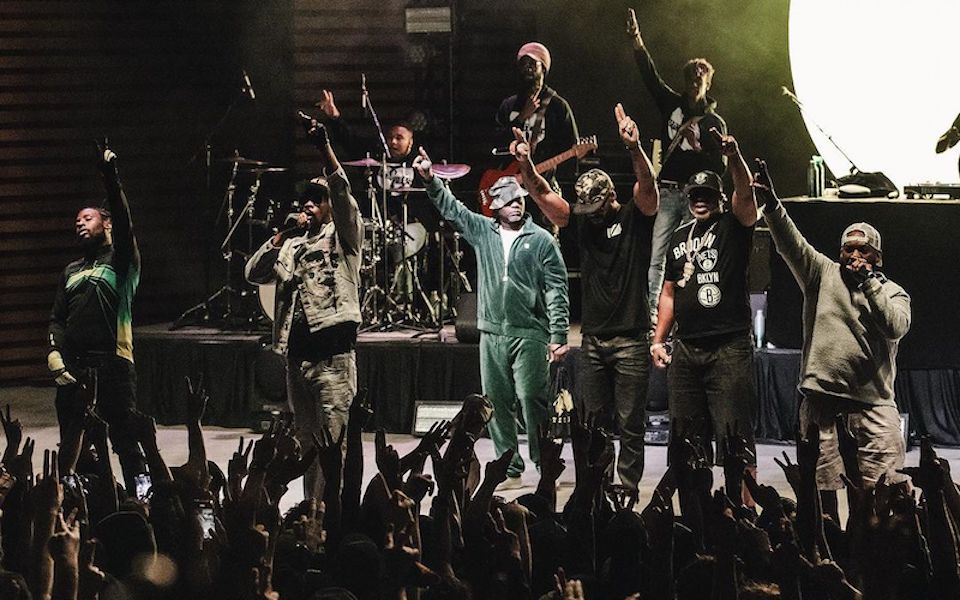In this photograph, taken from the perspective of a crowd member in an indoor stadium, we see a dynamic scene of a musical concert or performance. The stage is populated by a group of hip hop artists, and the image captures a moment of unified gesture, with each performer raising an arm into the air. In the foreground, there are six gentlemen in various stylish black outfits, their attire accented with unique details. Notably, one artist in the center stands out in a teal blue tracksuit. To the left, a performer in a dark outfit with green accents raises his left hand. Next to him, another in a white denim jacket and pants, complemented by a black undershirt and black sunglasses, also lifts his left arm. A performer in an all-green outfit with a white undershirt follows, while the next individual sports a black t-shirt, leather pants, and a black and camouflage hat. To his left, another artist wears a black shirt with "Brooklyn" and the number eight in white text, paired with black pants and a black hat featuring white text, raising his left hand in a peace sign. The artist on the far right is dressed in all-gray, including his hat, and raises his right hand in a peace sign as well.

In the background, there is a drummer on the left with his large drum set, extending his arm upward, and two guitar players on the right. One guitarist has one finger pointed near his chest, while the other has two fingers pointed up. The light gray stage is illuminated by a large white light in the top right corner. The audience below is engaged, many with their arms raised, mirroring the performers’ gestures, some throwing peace signs or rock-and-roll signs. Hints of the sound mixing area are visible in the top right, completing this vibrant and detailed depiction of the lively concert scene.